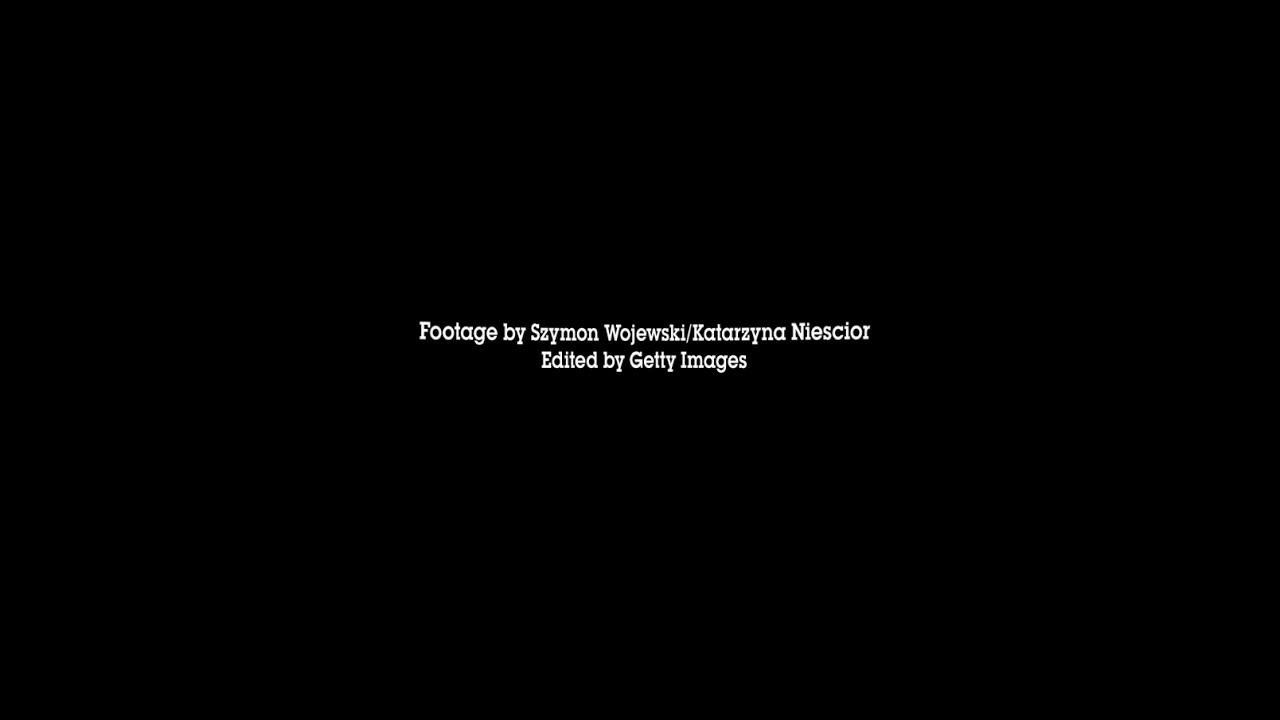The image features a pitch-black background, with a centered text caption in a tiny serif font, making the text difficult to read. The white text is arranged in two lines: the first line reads "footage by Szymon Wojewski / Katarzyna Nieskior" and the second line reads "edited by Getty Images." The overall appearance is reminiscent of the beginning or ending credits of a TV show or movie. There are no other graphics or additional text elements present in the image.